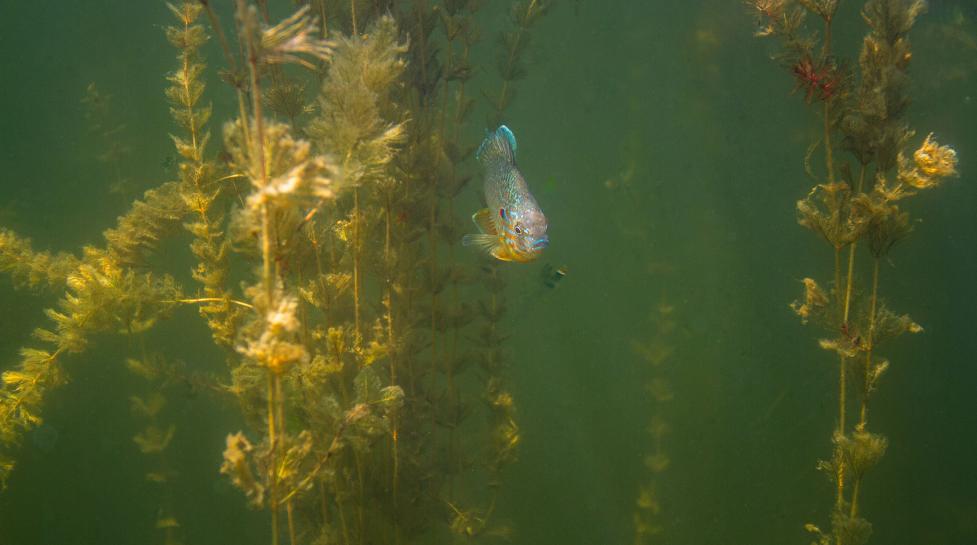In this horizontally aligned, underwater photograph, a small to medium-sized, colorful fish is prominently positioned in the center against a backdrop of murky green water. The fish, of an unidentified species, is a striking blend of colors: it possesses a neon blue upper part and a golden yellow lower part, with speckles of neon hues across its body. Notable features include a blunt nose, a large dorsal fin, and a blue line running above its mouth. The front and top view of the fish reveals a brownish silver-grey head merging into the vivid blue and yellow body, with additional blue trim on its fins. The scene is set amidst aquatic plants rising from the bottom of the frame, with long, slender stems and green leaves, some crossing over one another. There's also a hint of red coloration among the plants near the top right, perhaps a leaf or flower. The water is cloudy green, adding to the image's slightly blurry appearance, but the fish remains the focal point.